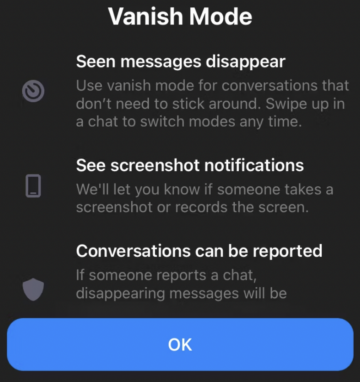This image is a screenshot of a mobile app settings page detailing the features of "Vanish Mode" in a chat application. The page has a sleek, square design and a dark background, either gray or black. At the top, it says "Vanish Mode" in bold white text. Below this heading, several options and descriptions are listed:

1. **Scene Messages Disappear**: "Use Vanish Mode for conversations that don't need to stick around. Swipe up in a chat to switch modes anytime." This option explains how messages will disappear after being viewed.

2. **See Screenshot Notifications**: Accompanied by an icon of a smartphone, the text states, "We'll let you know if someone takes a screenshot or records the screen." This feature notifies users if someone captures the chat.

3. **Conversations Can Be Reported**: This option has a gray badge icon next to it. The description indicates, "If someone reports a chat, disappearing messages will be..." (text possibly cut off in the screenshot).

The layout uses predominantly white and gray text, with gray icons for a clean and modern look, consistent with app interfaces rather than computer screens. There is a blue "OK" button at the bottom of the page for users to confirm and exit this settings overview.